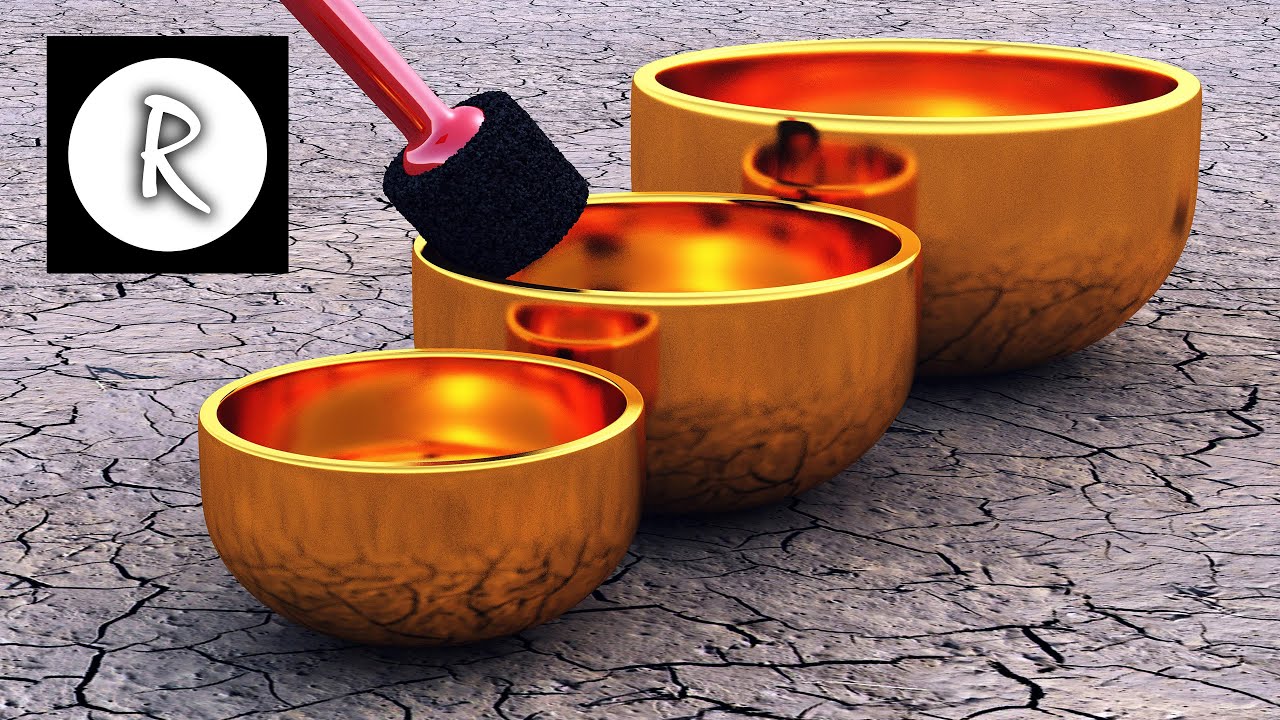The image is a computer-generated depiction of three highly reflective, golden-colored singing bowls arranged sequentially from smallest to largest. The smallest bowl is at the front, followed by the medium-sized bowl in the middle, and the largest bowl at the back. The bowls sit on a gray, cracked surface resembling drought-stricken ground, with the dark cracks clearly visible. The middle bowl features a brush with round black bristles and a shiny pink handle resting on it. In the upper left corner of the image, there is a black square logo containing a white circle and a black letter 'R' with a shadow effect. The reflective nature of the bowls captures the details of the surrounding surface and the overall ambient lighting suggests an overcast sky.